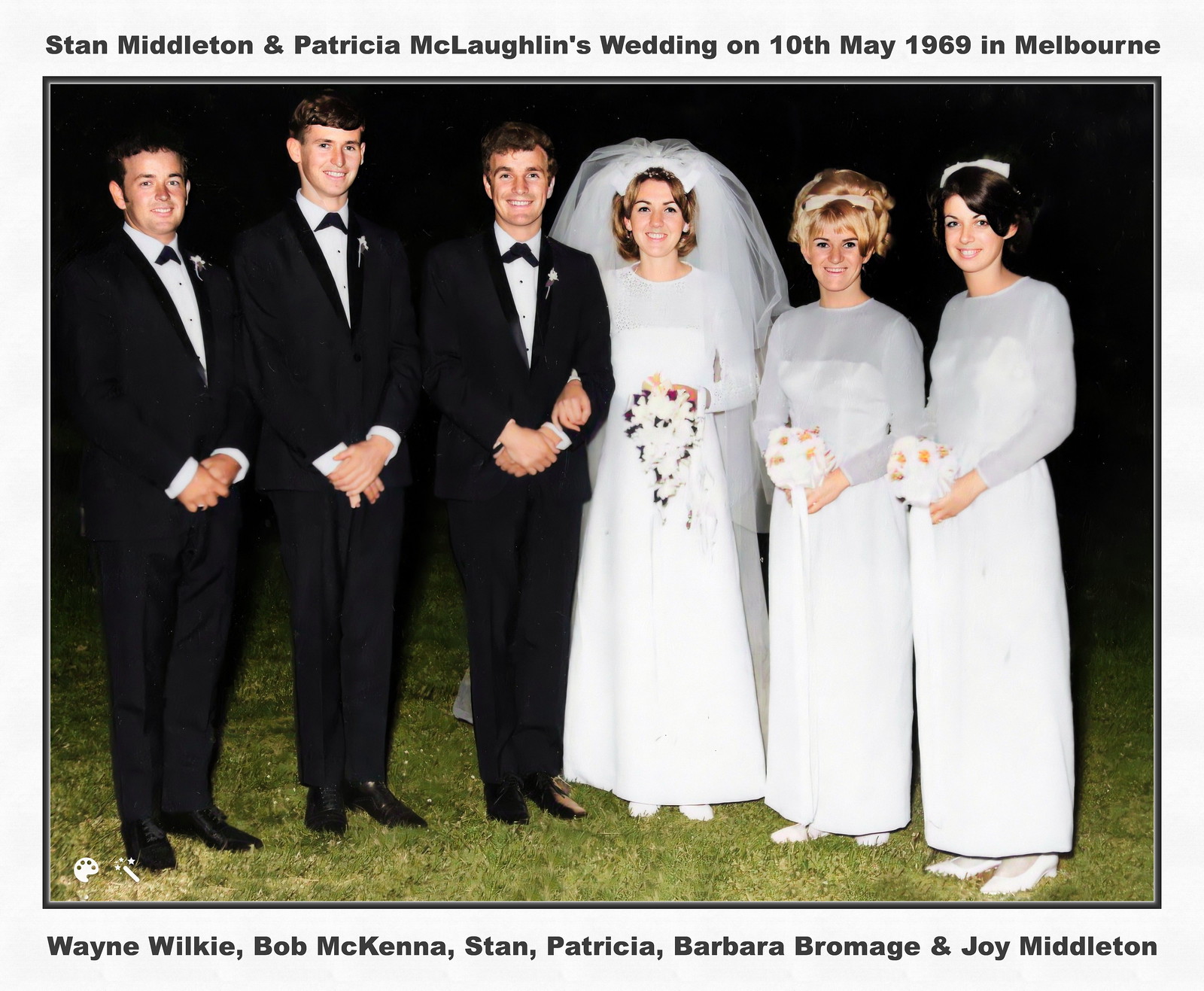The photograph features an elegantly detailed scene framed by a gray border. At the top of the image, text reads, "Stan Middleton and Patricia McLaughlin's Wedding on 10th May 1969 in Melbourne." Below, the names "Wayne Wilkie, Bob McKenna, Stan, Patricia, Barbara Bromage, and Joy Middleton" are printed, identifying the individuals present.

Centrally positioned in the image, six well-dressed people—three men and three women—stand on a grassy field. The men wear suits, and the women are adorned in dresses, reflecting the formal nature of the occasion. The colors in the image include shades of gray, black, white, green, yellow, orange, red, and pink, highlighting the diverse attire and vibrant setting.

This outdoor scene, seemingly captured at night, portrays the joyous ambiance of a wedding. The careful arrangement of the individuals and the detailed surroundings emphasize the significance and celebratory atmosphere of Stan and Patricia's special day.